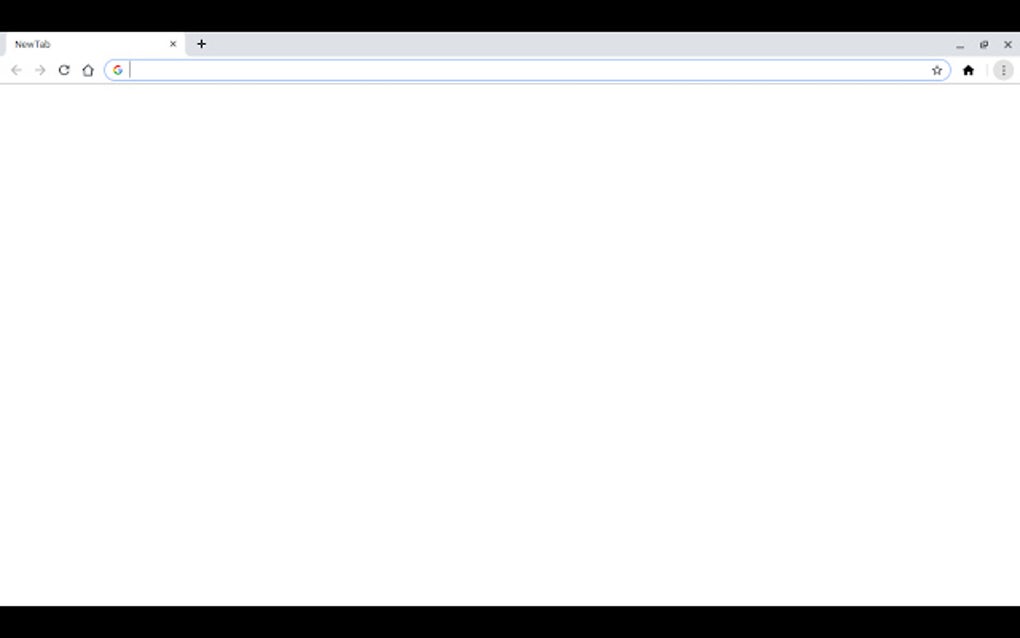The image shows a browser window with black borders at the top and bottom of the screen. On the left-hand side of the top border, there is a white tab labeled "New Tab" in small black font with capitalized "N" and "T." Adjacent to this tab is a small black "X," followed by a black plus sign on a gray background. To the right side of the top border is a gray underscore line, a box icon representing a window, and another "X" icon for exiting. 

Below this, two arrows point to the left and right respectively, followed by a refresh arrow that forms a circular shape. Next to the refresh arrow is a black house icon, symbolizing the home button. 

In the center of the toolbar is a search box. The search box is white on the inside and blue on the outside, featuring a multicolored Google "G" logo, with red at the top, followed by yellow, green, and blue sections. No text is present within the search box. 

On the far right of the search box, there is a thin vertical gray line, and further to the right, a red star icon with a white star in the middle, symbolizing bookmarks. Next to the star is a black home tab. Another vertical gray line separates this from a gray circular icon containing three horizontal gray lines. This circular icon represents the browser menu, with the three lines stacked one on top of the other.